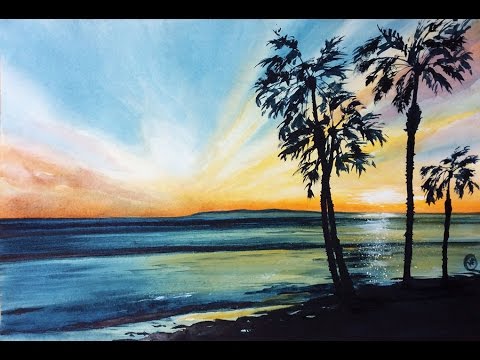This serene image, likely an oil painting, captures a tranquil tropical sunset. The picture is bordered by a black frame at the top and bottom. In the background, the sky shades from a deep blue at the top, transitioning through light blue and wispy clouds to a gradient of bright orange and pink near the horizon. The sun is setting in the lower right of the image, casting a warm reflection on the calm, shimmering water that stretches into the distance, where a small island shape can be seen. The ocean is a light blue near the shore, darkening towards the horizon. In the bottom right corner, there is a dark beach, appearing almost black due to the twilight. Four palm trees are silhouetted against the sky: two are intertwined, one stands alone, and another smaller one is positioned at the edge of the beach. The entire scene exudes a peaceful, end-of-day beauty, with delicate touches of light contrasting against the darkened elements of the landscape. There are also some unreadable initials in a circle on the right side of the image, adding a touch of mystery.